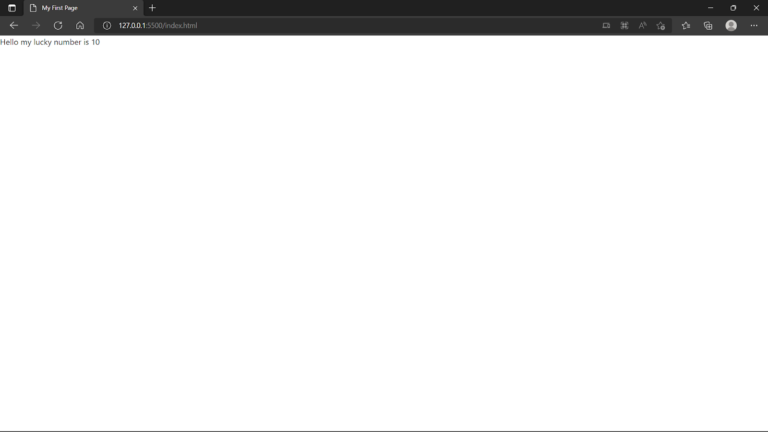The image is a horizontally rectangular screen capture of a computer interface. At the very top, there is a black horizontal banner divided into two sections. The top left corner of the banner displays a tab labeled "My First Page," accompanied by a plus icon for adding new tabs. On the far right, standard window control icons are visible, including minimize, expand, and close buttons.

The second section of the black banner contains navigational icons on the left side: back, forward, refresh, and home buttons. Adjacent to these icons, an address bar displays the URL "127.0.0.1:5500/index.html." To the right of the address bar, there is a less distinct cluster of icons that are too blurry to decipher clearly.

The main content area of the frame is predominantly white. In the upper left corner, there is a single line of text that reads, "Hello, my lucky number is 10."